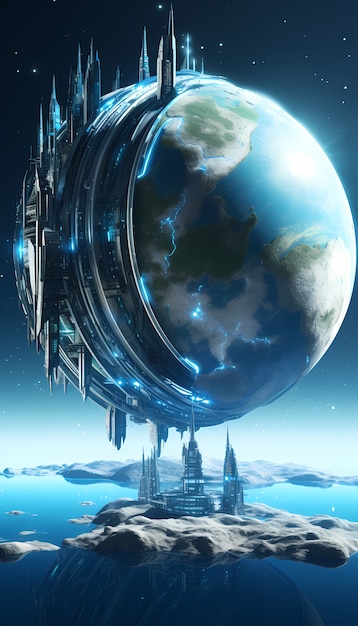The digitally created image, possibly AI-generated, depicts a large globe resembling Earth, floating centrally amidst a dark-to-light blue gradient background that transitions from space filled with tiny star-like white speckles at the top to lighter blues at the bottom. The planet is predominantly blue and gray with beige and green landmasses, encased in a futuristic metallic structure adorned with spiky skyscrapers and towers both above and below. These sharp, pointed buildings exude an advanced, high-tech aesthetic. Accompanying the globe's suspended appearance is an island-like base directly below, featuring a castle or futuristic building with similar pointed towers. This entire structure is surrounded by a blue water body, enhancing the science fiction ambiance. Additionally, subtle bluish glows suggest electrical currents running through the metallic casing, amplifying the high-tech, otherworldly vibe of the scene.